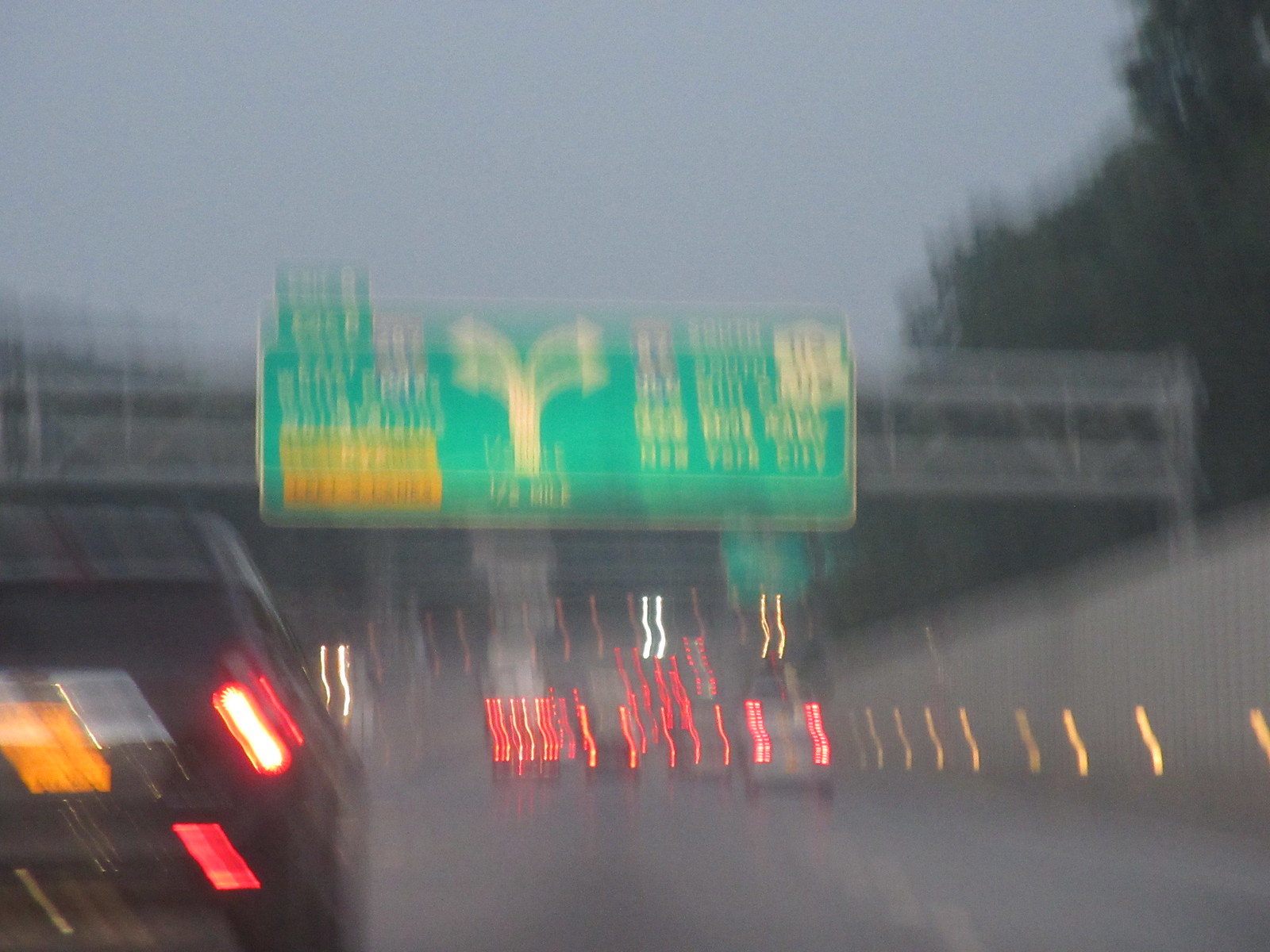The photograph presents a horizontally extended view of a highway scene, predominantly blurred, with a central focus on a large, green highway sign. The sign, which is positioned above what appears to be a silver and gray overpass, stands out against a gray sky backdrop. The overpass, though indistinct, displays a diagram of the road's split with white arrows directing traffic both to the right and to the left. Two numerical indicators are present on the sign, resembling typical highway route numbers, although they are not clearly legible. Below the overpass, there is blurred imagery of vehicle lights, predominantly red, indicating cars moving in the same direction. To the far left, there are one or two lights that suggest possible oncoming traffic, adding to the dynamic yet vague depiction of the scene.